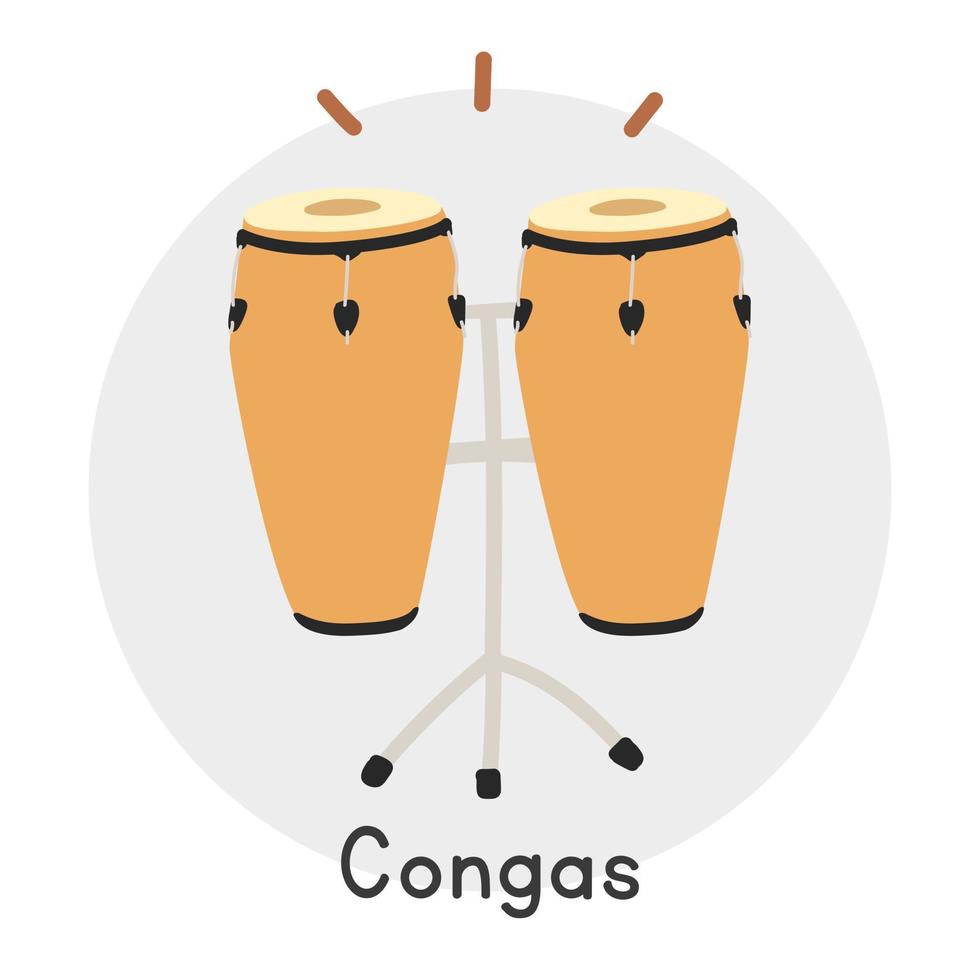This is a close-up illustration of two conga drums mounted on a light gray, three-legged stand against a light blue background. The congas are light brown with black bands around their tops and a cream-colored drumhead that features a central brown dot. The bottom of the image displays the word "congas" in black, with a capital "C" followed by lowercase letters. At the top of the illustration, three dark brown lines suggest vibrations or sound waves emanating from the drums. The entire scene is encapsulated within a light gray circle.